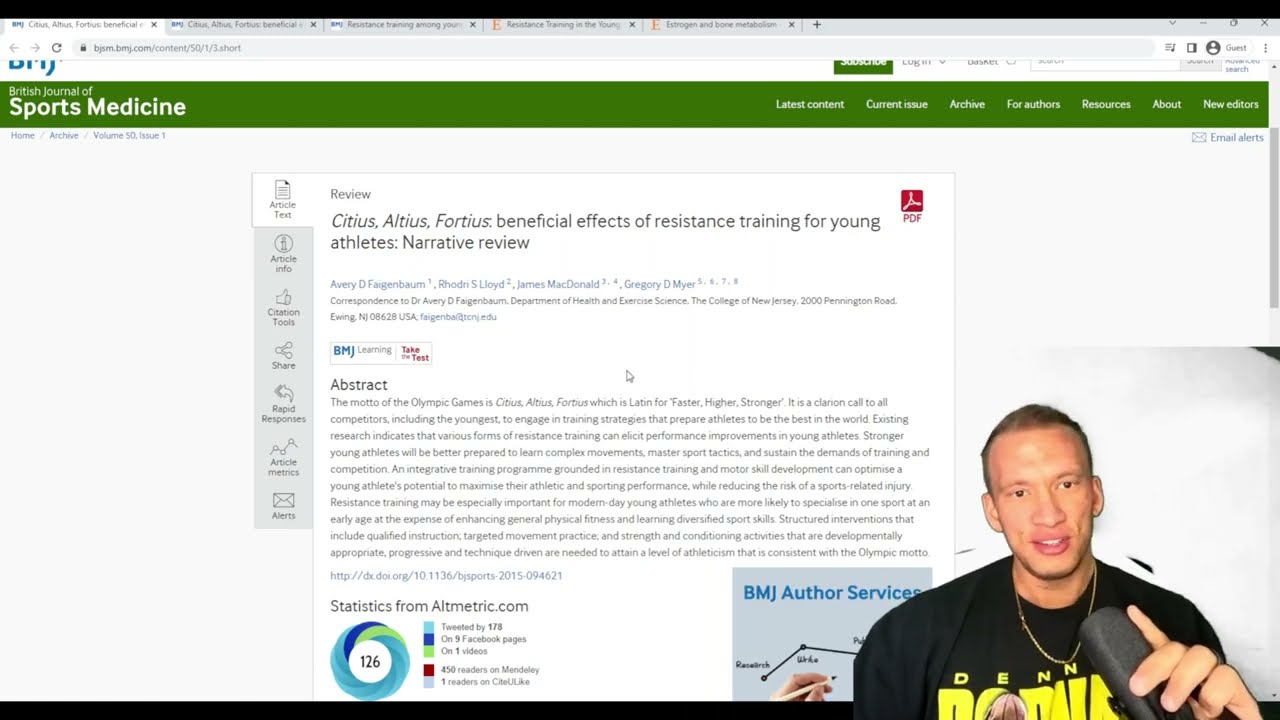The image captures a detailed screenshot of a sports medicine web page, prominently displaying a freeze-frame from a video presentation. Positioned in the bottom right corner of the webpage overlay is a man in his late 20s to early 30s, with short hair, wearing a black t-shirt featuring yellow text that likely reads "Dennis Rodman" along with a basketball graphic. The man accessorizes with a gold necklace and holds a microphone in his left hand, looking directly at the camera, possibly standing in front of a green screen.

The web page behind him is predominantly white and gray with a green banner at the top, displaying the title "Sports Medicine" in white text. The navigation menu, including options like "Latest Content," "Current Issue," "Archive," "For Authors," "Resources," and "About New Editors," runs along the top. The main article visible on the page is titled "Cyteus Alteus Forteus: Beneficial Effects of Resistance Training for Young Athletes, Narrative Review" in black text on a white background, accompanied by an abstract beneath it.

The overall composition suggests the man is discussing the content of the web page, highlighting its features and possibly the specifics of the journal article. Additional elements on the page include a graphic with statistics from altmetric.com and an illustration related to BMJ Author Services.